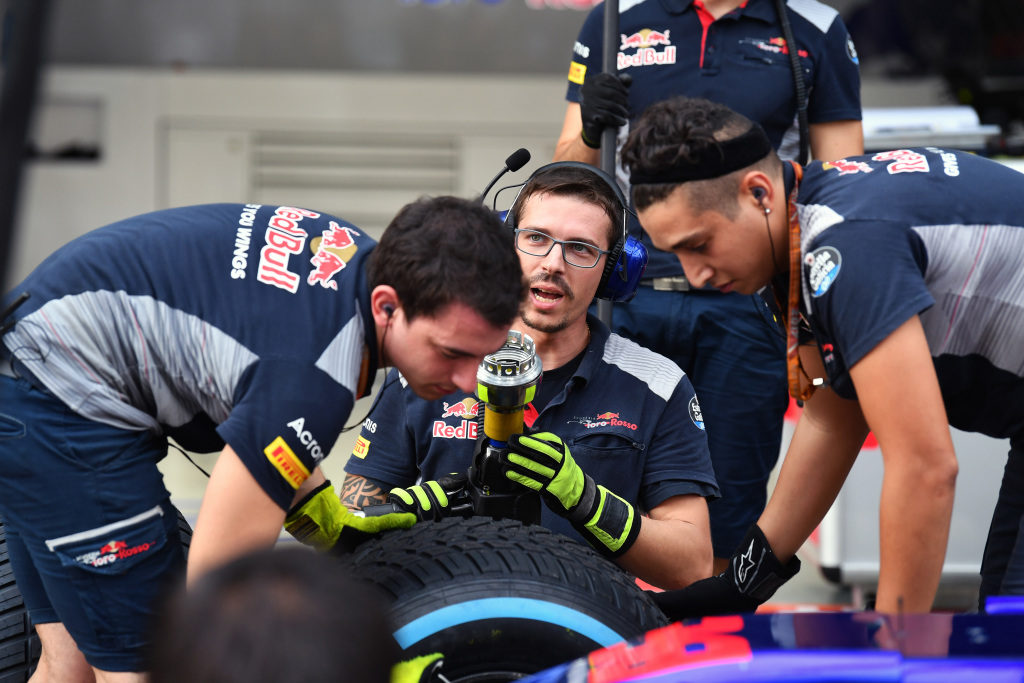The photograph captures a bustling pit stop scene likely involving the Red Bull Formula One race team. At the center, a man resembling a news broadcaster is seated, sporting blue headphones, blue glasses, and green-and-black gloves, and he wears a sponsored t-shirt emblazoned with the Red Bull logo. To his sides, two other men in matching uniforms — blue and grey shirts with "Red Bull gives you wings" on the back, and blue shorts — are in the process of changing a tire. One of them wears a black headband and has a device in his ear, indicating coordinated communication. They are using various tools, including one designed to rapidly unscrew or screw the tire. In the blurry background, another man in the same outfit, but without a visible head, holds an instrument possibly used for lifting the car. The chaotic energy, shared focus, and array of colors — red, white, blue, grey, black, and several shades of yellow — suggest a high-stakes moment during the race, all contributing to the vivid scene of a pit crew hard at work.